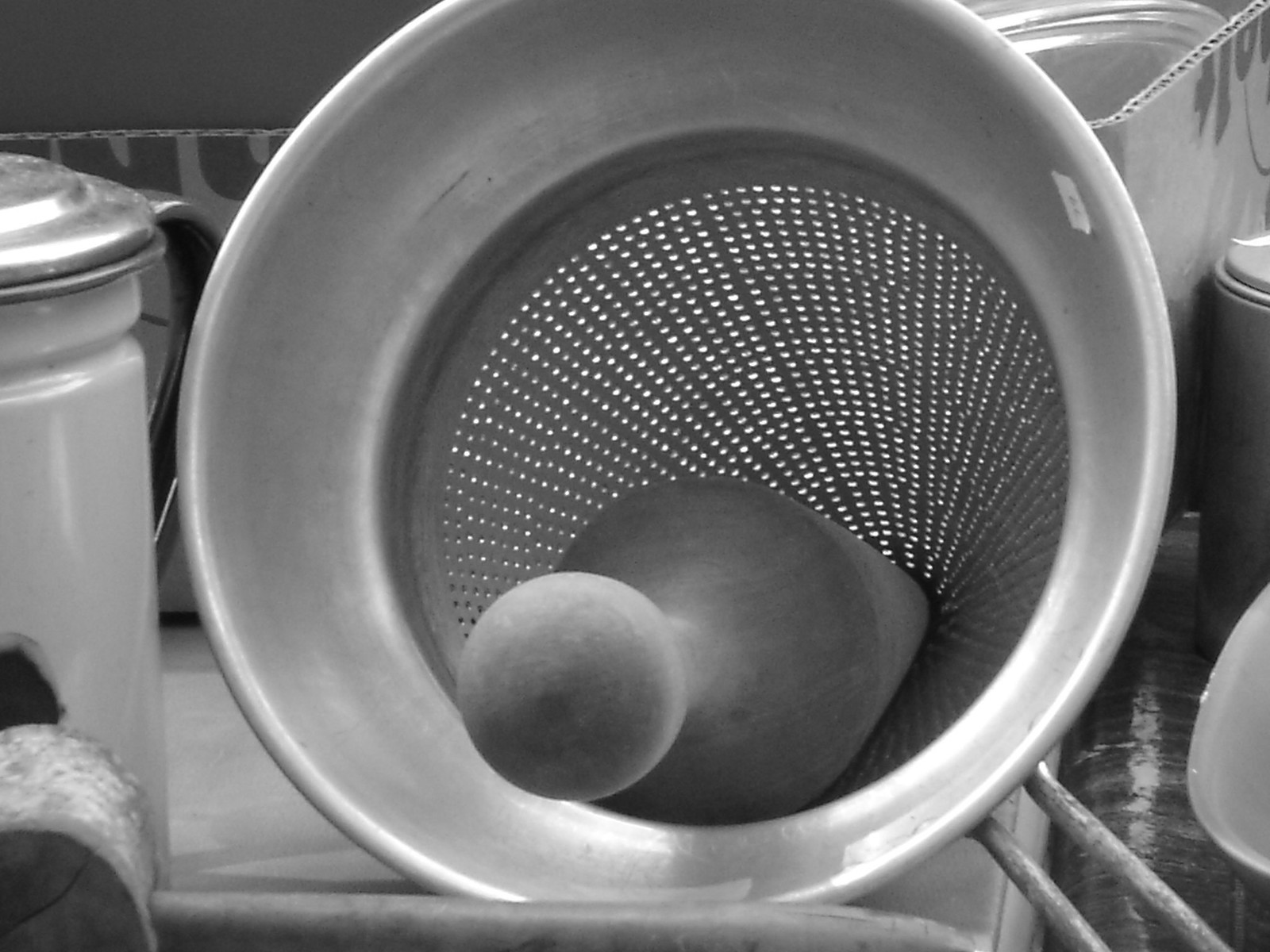The black and white photograph, set in a kitchen, prominently features a large metal colander lying on its side on a white countertop. The colander, which has a solid lip at the top and a cone-shaped base with holes, includes a small wire handle visible at the bottom right. Inside the colander, there is a wooden plug or pestle, suggesting it could be used for mashing vegetables and allowing juice to run out while retaining the pulp. Surrounding the colander, to the left, there is a white pitcher with a lid and a handle. On the right, there are several containers, including a jar and a small box with an unclear silver lid. Additionally, there is a wooden mallet resting on the countertop near the colander. The overall scene is a detailed view of various kitchen utensils arranged around the central colander, emphasizing its potential use for food preparation.